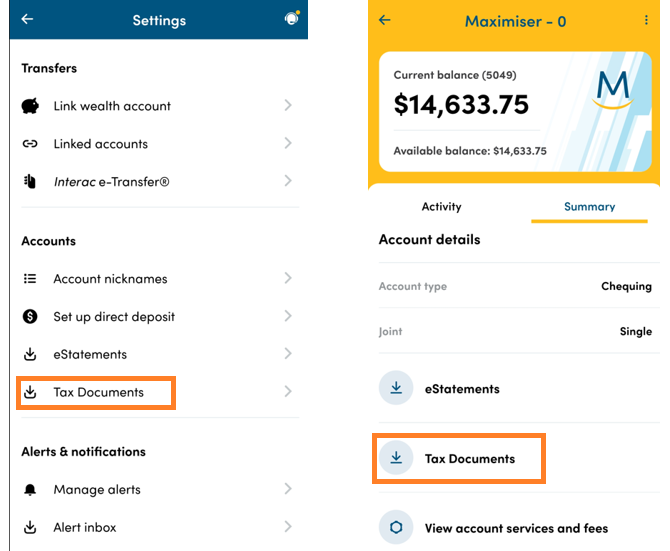Here are two detailed screenshots showcasing the user interface of a phone's banking app settings and account overview pages. 

**First Screenshot:**

- The settings page is displayed with a white background and features a prominent blue bar at the top. The blue bar has the title "Settings."
- Below the settings title, there are numerous sections listed:
  - "Transfers," "Link Wealth Account," "Linked Accounts," and "Interac Transfer."
  - A section titled "Accounts," which includes options such as "Account Nicknames," "Set Up Direct Deposit," "E-Statements," and "Tax Documents." The "Tax Documents" option is highlighted in orange for emphasis.
  - At the very bottom, it displays "Alerts and Notifications," which contains sub-options like "Manage Alerts," and "Alert Inbox."

**Second Screenshot:**

- The top section contains an orange rectangular banner with a white inner rectangle that displays the "Current Balance" of $14,633.75 in bold text. 
- Directly beneath the current balance are two buttons: "Activity" and "Summary." The "Summary" button is currently selected.
- The "Summary" section provides detailed account information, including:
  - "Account Details," specifying the "Account Type" as Checking, Joint, or Single.
  - Three buttons for different functionalities: "E-Statements," "Tax Documents," and "View Account Services and Fees."
- The "Tax Documents" button is highlighted with an orange rectangle, and a download icon (an arrow with a line) is adjacent to it.
- Similarly, the "E-Statements" button also features a download icon next to it.

This comprehensive presentation of the two screenshots highlights various options and functionalities available within the banking app, providing clear guidance on where to find specific features such as tax documents and account services.